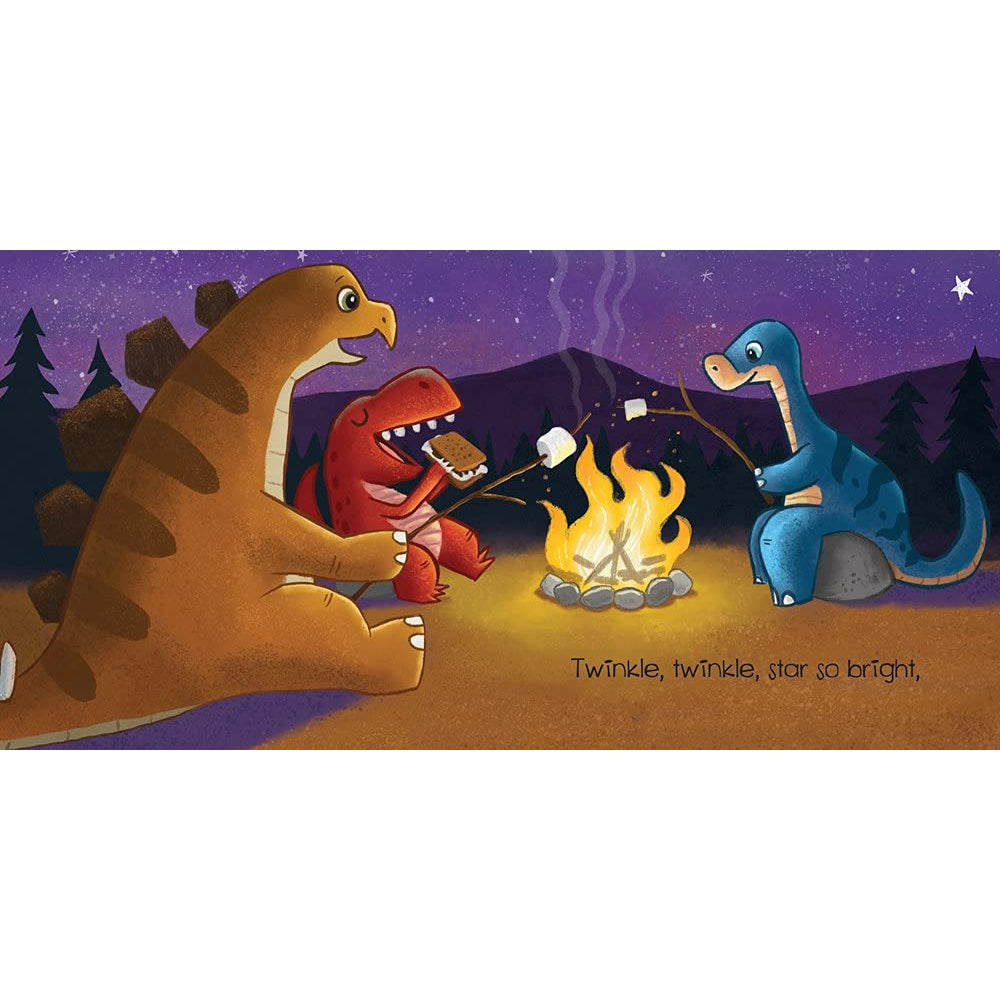In this horizontally-oriented cartoon image, three dinosaurs are gathered around a campfire on a nighttime camping scene. The sky, rendered in various shades of purple, is dotted with stars, including one larger star in the upper right corner. The campfire, glowing with yellow and white flames, is situated slightly to the right of center, encircled by gray rocks and topped with sticks.

To the left, a yellowish-brown stegosaurus with brown stripes sits on its haunches, holding a stick with a marshmallow over the flames. In the middle, furthest from the viewer, an orange dinosaur enjoys a s'more, displaying its brown stripe. On the right, a blue dinosaur with darker stripes roasts a marshmallow while seated on a rock. The scene is set against a backdrop of mountains and scattered pine trees, shrouded in the purple night sky. At the bottom of the image, a caption reads, "Twinkle, twinkle, star so bright."